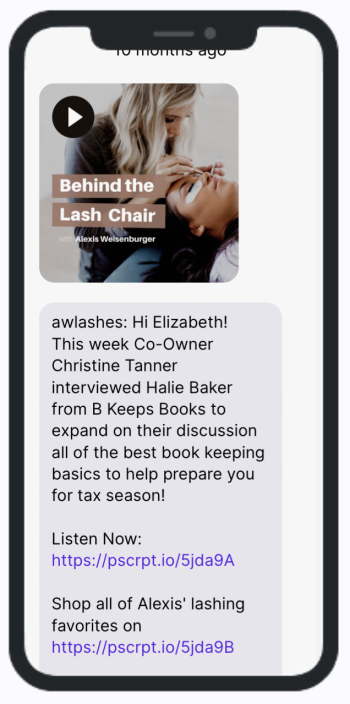Image Caption:

"A black-outlined image resembling a cell phone highlights a video thumbnail at the top. The thumbnail shows a blonde woman performing an eye or eyelash procedure on another woman who is lying down with stickers beneath her eyes. An arrow indicates a playable video feature. Inside the image, text reads, 'AW Lashes. Hi Elizabeth! This week, co-owner Christine Tanner interviewed Haley Baker from Bee Keeps Books to expand on their discussion of the best bookkeeping basics to help you prepare for tax season. Listen now.' Below this, there is a clickable purple link. Additionally, another message reads, 'Shop all of Alexis' lashing favorites,' followed by another clickable purple link: https://pscrpt.io/-5JDA9B."